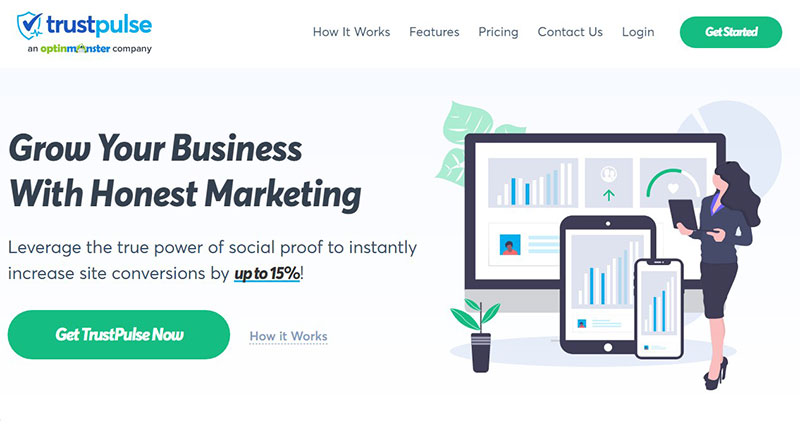The image is a promotional graphic from a company called Trust Pulse. Across the top, there is a navigation bar featuring tabs labeled "How It Works," "Features," "Pricing," and "Contact Us," with a login option available as well. Prominently displayed is a green button that says "Get Started." 

The top of the image includes a bold headline that reads, "Grow your business with honest marketing," followed by a subtext that states, "Leverage the true power of social proof to instantly increase site conversions by up to 15%."

At the bottom of the image, there is another green, rectangular button with curved edges that says "Get Trust Pulse Now." To the immediate right of this button, there is a small-print phrase, "How it works."

To the right side of the image, we see a stylized illustration of a businesswoman. She is depicted wearing a suit jacket and skirt, accessorized with black high heels. It is important to note that this is a digital drawing, not a real photograph. The businesswoman stands in front of a digital board, and she is holding a tablet, akin to an iPad, in one hand and a phone in the other.